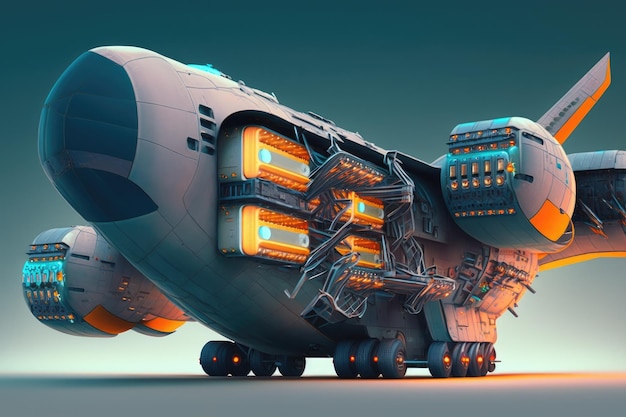This high-definition, modern illustration showcases a futuristic aircraft that seems more at home in a science fiction movie than in real life. The plane, predominantly gray with trim in yellow and orange, features an exploded open side, revealing two floors of passengers, and various internal components that resemble stylized cassette tape decks. The aircraft's body is large, squat, and oblong, with three rows of three wheels on each side, each wheel featuring an orange-yellow lit center. The detailed illustration also highlights several round, well-lit objects next to the wings, which might function as storage areas, and an array of exposed wires and power supplies. The tail fin is just barely visible and carries some obscured lettering. While the plane lacks large windows, there are five small slots towards the front, along with an additional single slot ahead of them, accentuating its high-tech, modern design.